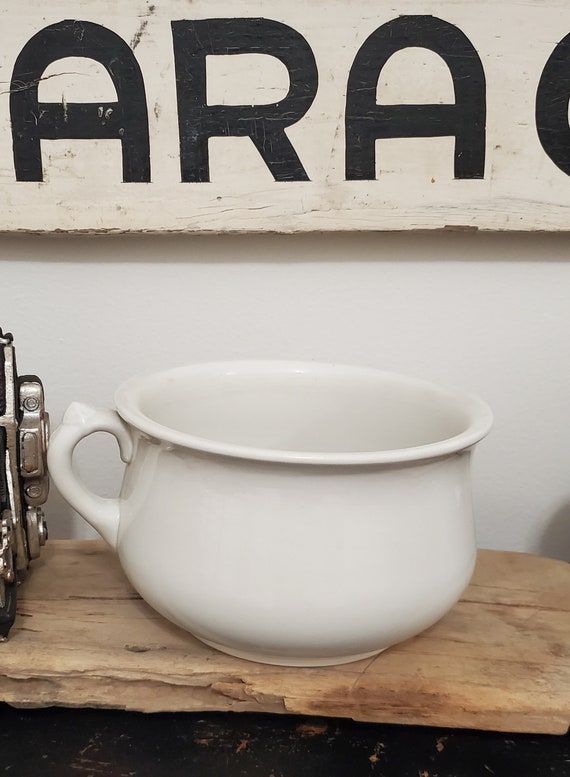This detailed photograph-like drawing depicts an indoor setting with a prominent white ceramic mug, possibly 8 to 12 inches wide, featuring a handle on the left side. The mug sits atop an inclined, unfinished wooden plank marred by gouges. The white wall behind the mug hosts a mounted white wooden sign that bears the bold black letters "A.R.A." There appears to be the partial letter "O" following these letters. To the left of the mug, a silver or steel-colored arm of an unidentified metal equipment peeks into the frame. The overall simplicity of the scene, combined with its elements, suggests a cozy, possibly café-like atmosphere. The image does not feature any people.